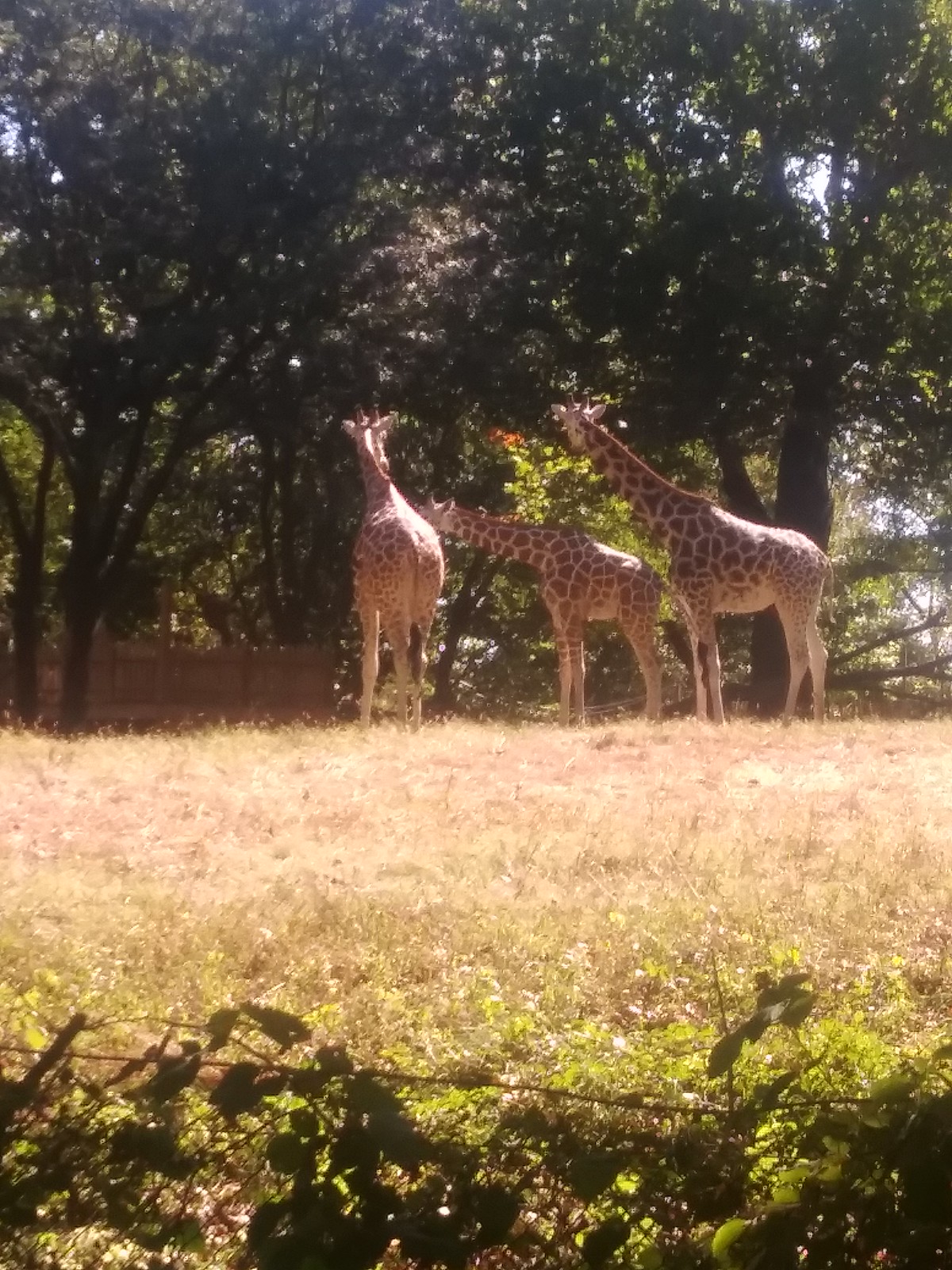This medium-resolution photograph, taken outdoors on a sunny day, features three giraffes situated across a grassy area, with a mix of brown and green hues, as well as some twigs and low-lying plants visible in the foreground. The photo, captured from a low angle, gives a sense of the ground's perspective. In the background, near some trees and partially obscured by wooden and small wire fencing, the three giraffes stand tall. The giraffe on the left is viewed from behind, displaying its back and hind legs as it faces the trees. The two giraffes on the right face the left; one has its neck extended horizontally, appearing to be eating leaves from the trees, while the other has its neck slightly lower. The closer giraffe to the right seems to glance towards the camera. Beyond the giraffes, patches of blue sky peek through the foliage, enhancing the midday sunlight that casts subtle shadows of leaves onto the grass below.